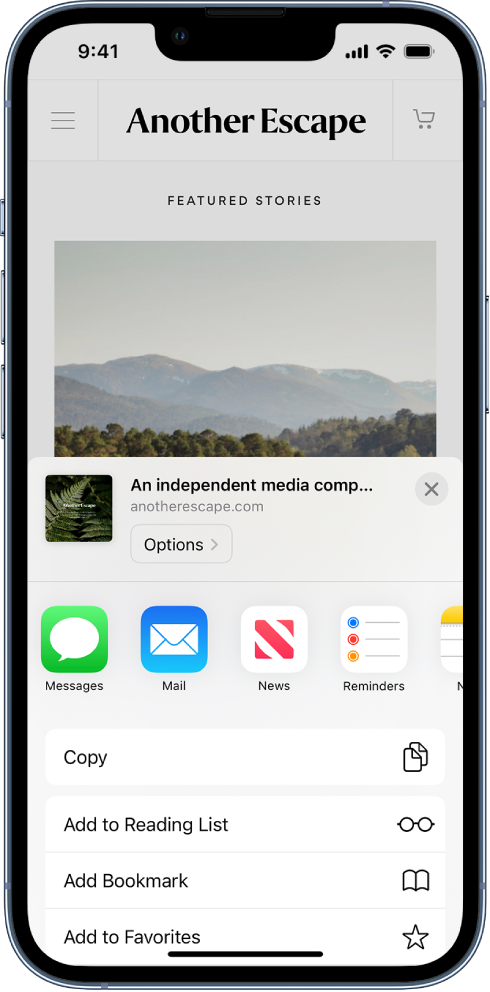This image depicts a stylized outline of a smartphone against a white background. The black outline resembles a functioning phone, showcasing various on-screen elements. At the top of the phone display, the time is indicated as "9:01" in black ink, alongside icons for battery status, network connectivity, and WiFi, all rendered in black on the white background.

The phone screen displays an open app, titled "Another Escape" in bold black text. To the left of this title is an options button, and to the right, a shopping cart icon. Below the app title, the section "Featured Stories" is prominently featured, accompanied by a picturesque image of a serene mountain and tree landscape.

Further down, the caption "An Independent Media Camp" appears, accompanied by an additional image. The interface suggests options for sharing content via messages, email, news, and reminders. Additional functionalities include copying, adding to the reading list, bookmarking, or marking as a favorite. All text is meticulously presented in black ink, maintaining a clean and minimalist aesthetic.